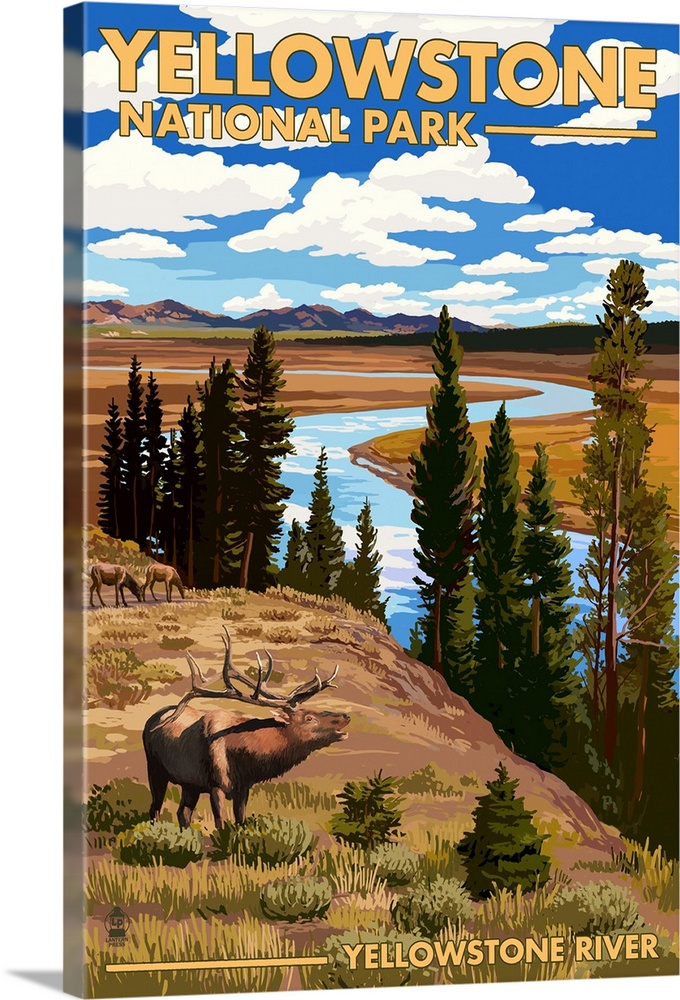This image is a canvas print mock-up depicting a scenic view of Yellowstone National Park. At the very top, in slightly blurred large yellow letters with black outlines, are the words "Yellowstone National Park." The word "Yellowstone" is double the size of "National Park," and the text sits against a blue sky filled with fluffy white clouds of varying shades.

The artwork features a vector-style scene that leans towards a photorealistic look without strong outlines. Dominating the bottom left of the image is an elk, with its mouth open as if bugling. The elk stands on a grassy hill, facing right, with prominent antlers visible. Surrounding the elk is lush grass, and behind it, tall trees line the hill.

In the mid-background, a blue river winds gracefully, curving into the distance. This river is bordered by fern-like trees, creating a natural frame that leads the eye deeper into the landscape. Finally, the far background showcases a majestic mountain range, completing the picturesque scene designed to evoke the beauty and wilderness of Yellowstone National Park.